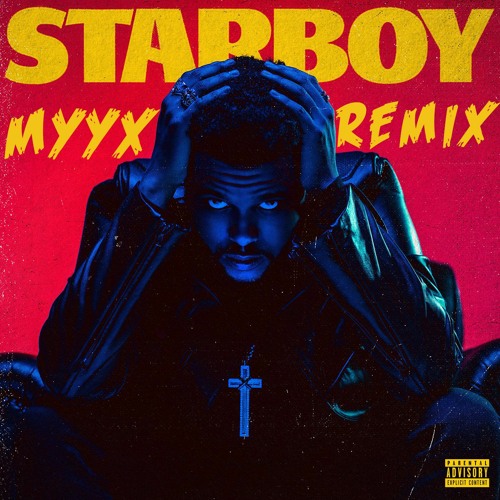This striking album cover for "Starboy MYYX Remix" features a red background with bold yellow lettering. At the top, the title "Starboy" is prominently displayed, followed by "Mix" on the left, "MYYX" in the center, and "Remix" on the right. In the bottom-right corner, a yellow and black "Parental Advisory Explicit Content" label is prominently placed. The focal point of the image is a man, The Weeknd, drawn in detailed black and blue tones. He is seated indoors, leaning forward with his elbows resting on his knees and his hands covering his head. His fingers extend to the top of his head, creating visible creases in his forehead. Although his face is angled slightly downward, his piercing gaze is directed upward towards the viewer. The Weeknd is adorned with a large, illuminated blue cross around his neck that starkly contrasts against his black leather jacket, which features zippers on the sleeves. This vivid and intricate illustration captures a contemplative and intense atmosphere, emphasizing both the artist's cool demeanor and the album's bold design.